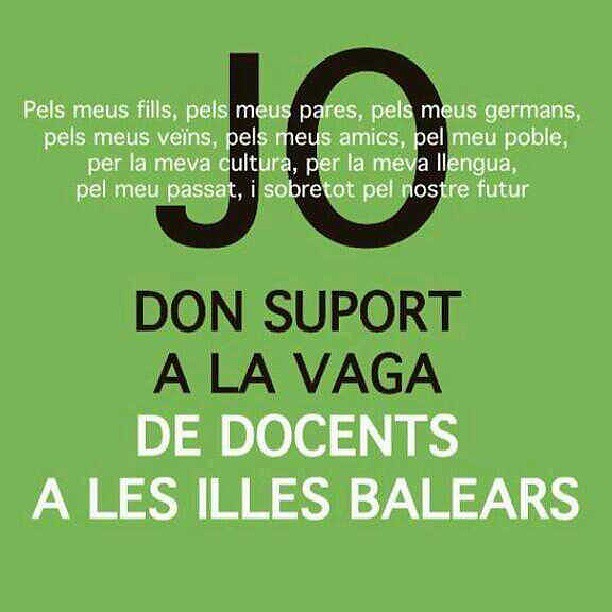The image depicts a medium green square sign with slight blue undertones, featuring text in an unidentified foreign language. Prominently at the top, there is a very large "J-O" written in black. Superimposed across the "J-O" are smaller, slightly blurred white letters forming a sentence that reads, "PELSMEUSFILLSPELSMEUSPARESGERMANSSPELSMEUSBELNSGERMANSSPELSMEUSAMICSPELMEUPOBLEPERLAEDUCULTURAPERLALENEGUAPERMEUPASSATISOBRETOTPELLOSTREFUTUR." Beneath the "J-O," in black text are the words "Don Supportala Vaga," followed by white block letters stating "Dedocents a la Iles Valliers." Each segment of text varies in size and placement, creating a visually detailed and intricate sign.